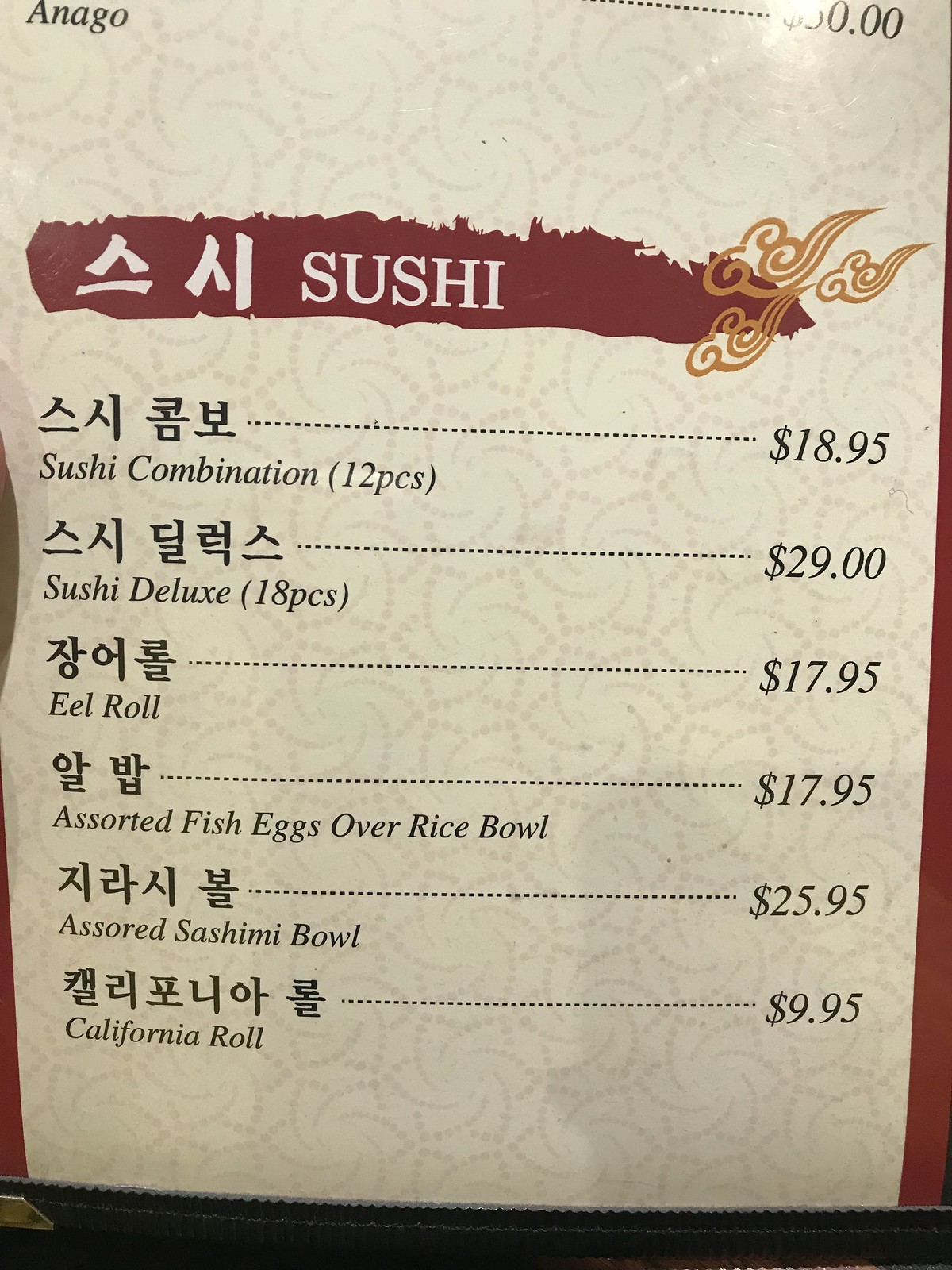This image depicts a page from a Japanese restaurant menu. At the very top, a red stripe features the word "Sushi" prominently in white letters. Below this heading, six different menu items are listed, each with a combination of English and Japanese text. The first item is a Sushi Combination consisting of 12 pieces priced at $18.95. Following this is the Sushi Deluxe with 18 pieces for $29. Next is the Eel Roll, priced at $17.95. Below that is an Assorted Fish Eggs Over Rice Bowl for $17.95. The menu continues with an Assorted Sashimi Bowl, which costs $25.95. Finally, the last item on the list is a California Roll, available for $9.95. This menu page is printed on an elegant off-white paper adorned with tan, swirly lines, giving it a sophisticated and upscale appearance.